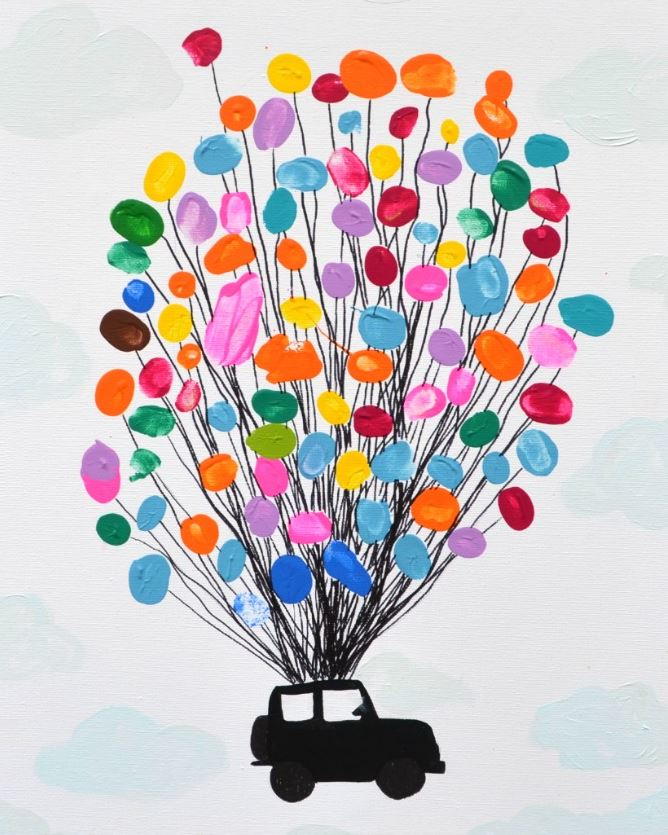This intricate abstract oil painting, displayed on a white canvas, features the distinct figure of a black vehicle resembling a Jeep or SUV. The car, depicted with minimal yet defining details such as two white windows, dark gray wheels, and a faint steering wheel, is the central focus. Emanating from its sunroof is a mass of 50 to 100 vividly colored balloons tethered by thin black strings, reminiscent of the iconic scene from the movie "Up." These balloons, painted in vibrant shades of blue, light blue, red, pink, green, dark and light green, orange, yellow, lavender, purple, and even brown, hover in the air as if lifting the car. The background of the painting, though primarily white, is accented with barely perceptible light blue clouds scattered throughout, adding a sense of whimsy and ethereal lightness to the piece. Overall, the dynamic composition of the floating black Jeep carried by an array of multi-colored balloons against a cloud-dotted white backdrop creates a captivating and dreamlike visual narrative.